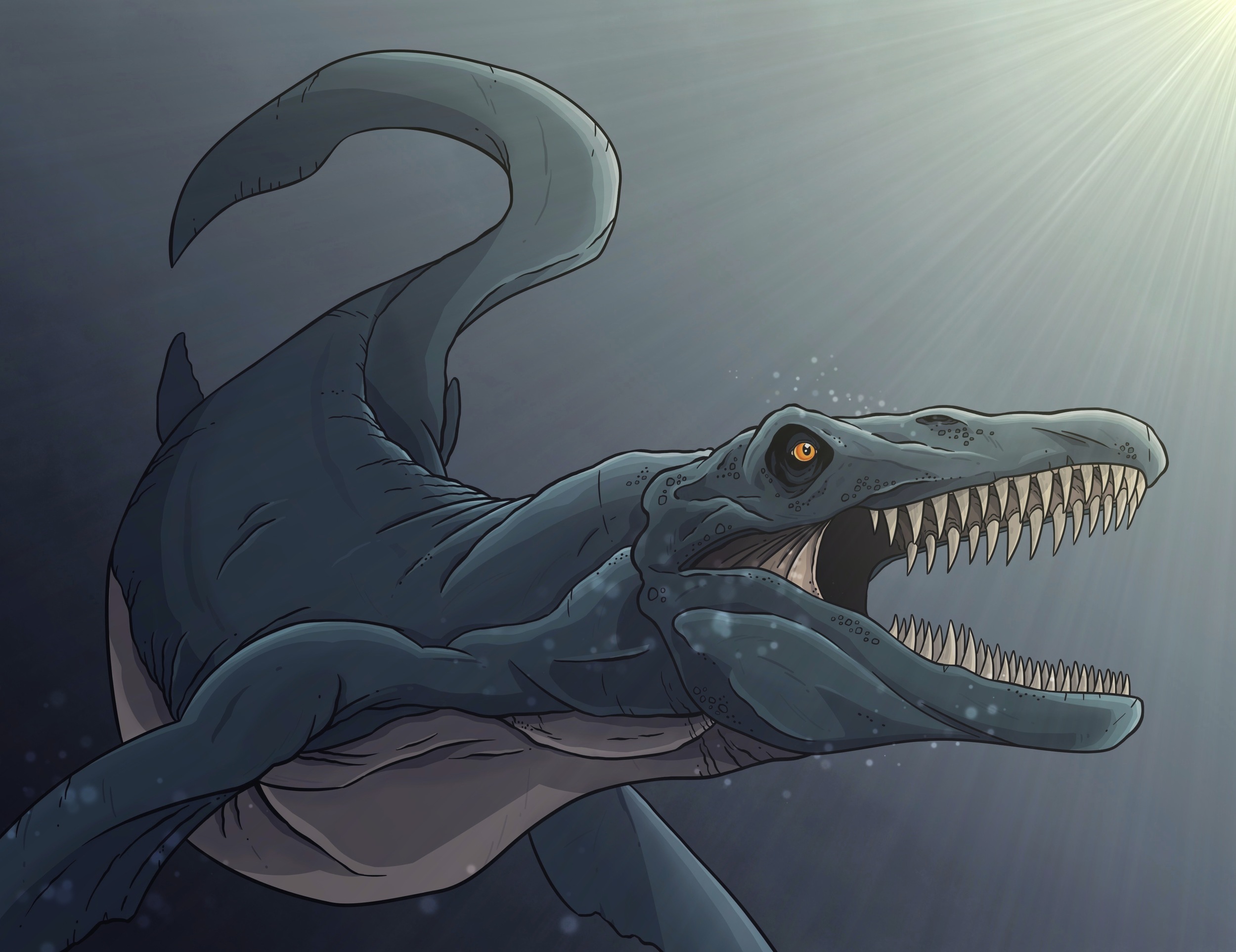The cartoonish image depicts an aquatic dinosaur swimming in the ocean, surrounded by a gray-blue underwater environment with bubbles, accentuated by rays of sunlight streaming from the top right corner. The dinosaur's head, reminiscent of a T-Rex with an orange-yellow eye, an oversized black pupil, and an open mouth brimming with sharp, white teeth, dominates the scene. Its body, seen from the left side, reveals a broad, gray-green hue on the upper side and a beige-gray underbelly. The creature's design includes a long, tapered tail, two front flippers with paw-like ends, and two additional flippers at the back. The entire portrayal captures the motion of the dinosaur swimming downward and turning in the aquatic setting reminiscent of the Loch Ness Monster.